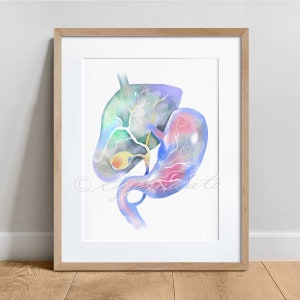The image depicts a framed piece of abstract art, photographed indoors against a light grey wall with a broad white trim at the base. The floor is a warm brown hardwood. The artwork, encased in a light brown wooden frame, presents an abstract representation of human organs, possibly elements of the digestive or respiratory system. The central forms suggest parts of the digestive tract, with vivid blue, red, orange, and white hues creating a striking, fluid-like depiction. The top left section features a blob shape tapering into a tube, which connects to a larger, lung-like structure marked with red and white hues. The frame's background is white, accentuating the dynamic color transitions from light green to dark green and yellow, to shades of light red and blue within the depicted organs. The image includes an indiscernible cursive watermark which appears to say "S-Z-Y-M-A-N art" or a similar variation, hinting at the artist's or photographer's signature. The overall composition carries a professional, somewhat medical yet abstract aesthetic, underscored by the fluid merging and blending of colors.